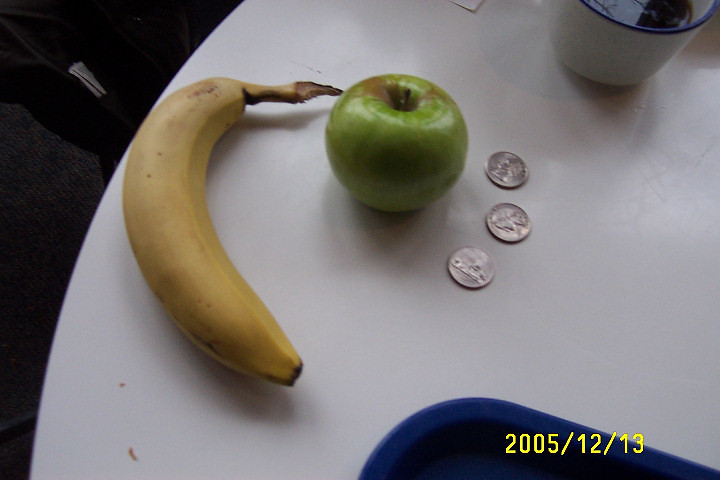This overhead shot captures a round white table that dominates most of the frame, with a shadowy black background in the top right corner. A white mug with a blue rim is placed in the top right section of the table, containing a dark liquid, likely tea or coffee. In the bottom right, a medium blue item, possibly a tray, sits partially visible. The centerpiece of the image is a vibrant green Granny Smith apple located almost exactly in the center of the table. To the right of the apple, three quarters are positioned in a slight curve. On the left side of the apple, an unopened banana, appearing semi-ripe, is placed with noticeable smudges or crumbs on its bottom right side. This clean and minimalistic scene offers a simple yet detailed arrangement of everyday items.